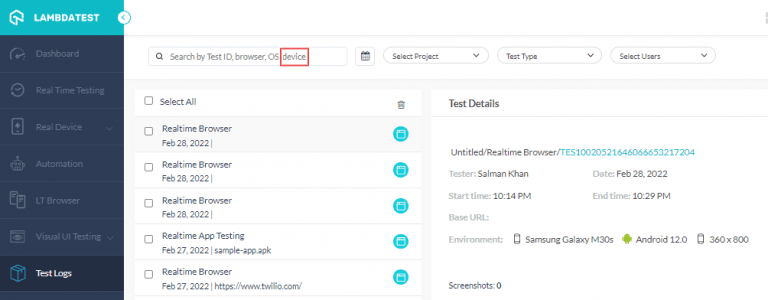This image is a screenshot of a computer interface for a web testing platform named LambdaTest. The screenshot is in a long, horizontal rectangular format.

On the left side of the screen, a vertical navigation menu is displayed on a blue background. This menu includes clickable options in darker blue that read: “Dashboard,” “Real-Time Testing,” “Real Device,” “Automation,” “LT Browser,” “Visual UI Testing,” and “Test Logs.” 

To the right of this menu is a search bar where users can search by “Test ID,” “Browser,” “OS,” or “Device.” In the screenshot, a red box highlights the “Device” option, indicating that the user is searching by device.

Further to the right are several dropdown menus labeled “Select Project,” “Test Type,” and “Select Users,” each with an accompanying down arrow for expanding the options.

In the central part of the image, there is a list titled with "Select All" and checkboxes beside options like “Real-Time Browser” and “Real-Time App Testing,” allowing users to select various testing types. Adjacent to these options are blue circular icons featuring symbols that resemble a computer or a clipboard.

On the right side of the screenshot is a section labeled “Test Details,” providing specific information about the test environment. The details mention a device, “Samsung Galaxy,” and an operating system, “Android,” with a resolution of "360 by 800," among other technical parameters. This section appears to summarize the specifics of the testing environment in use, although the exact nature of the data is not fully clear. 

Overall, the image captures the detailed interface of a web testing tool designed to manage and execute various testing scenarios on multiple devices and browsers.